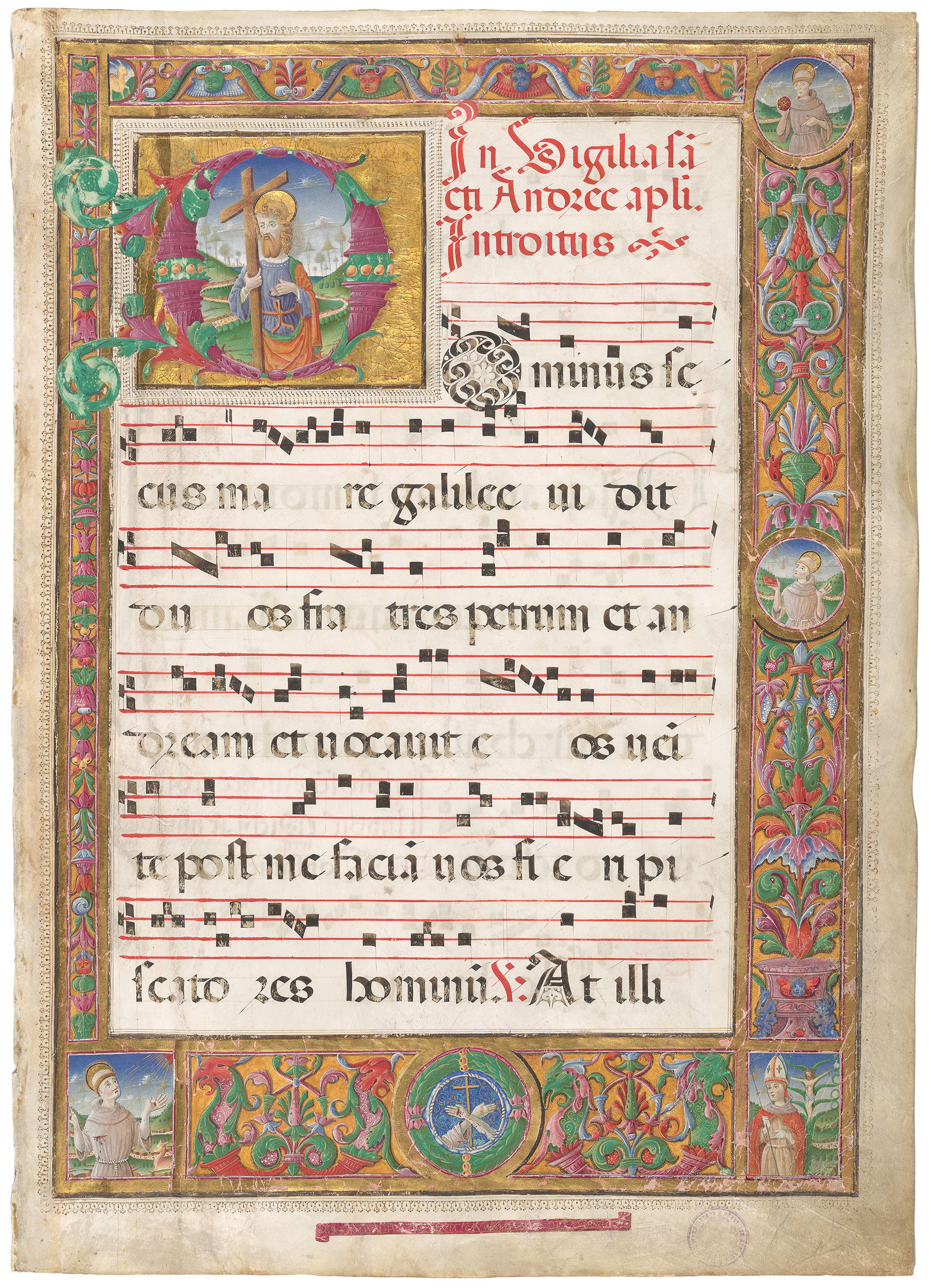This image showcases an exquisitely decorated piece of medieval-style music manuscript. The document is set on dark cream-colored paper, evidencing its age along the edges. The borders framing the music are intricate: the top and left borders are relatively thin, while the bottom and right ones are considerably thicker. These borders are adorned with vibrant jewel tones, including rich reds and greens, interspersed with floral motifs. Additionally, certain sections feature a striking blue, within which angelic figures are delicately illustrated.

Inside this ornate border lies a pristine white rectangle displaying the musical notation, with lyrics meticulously inscribed beneath in a Gothic font. Dominating the top left corner is a grand, golden “D,” set within a bold block, which contains an illustration of a figure, presumably significant to the text or music. This ornate initial and the surrounding embellishments bear testament to the era’s artistic devotion, effectively capturing the essence of medieval manuscript illumination.